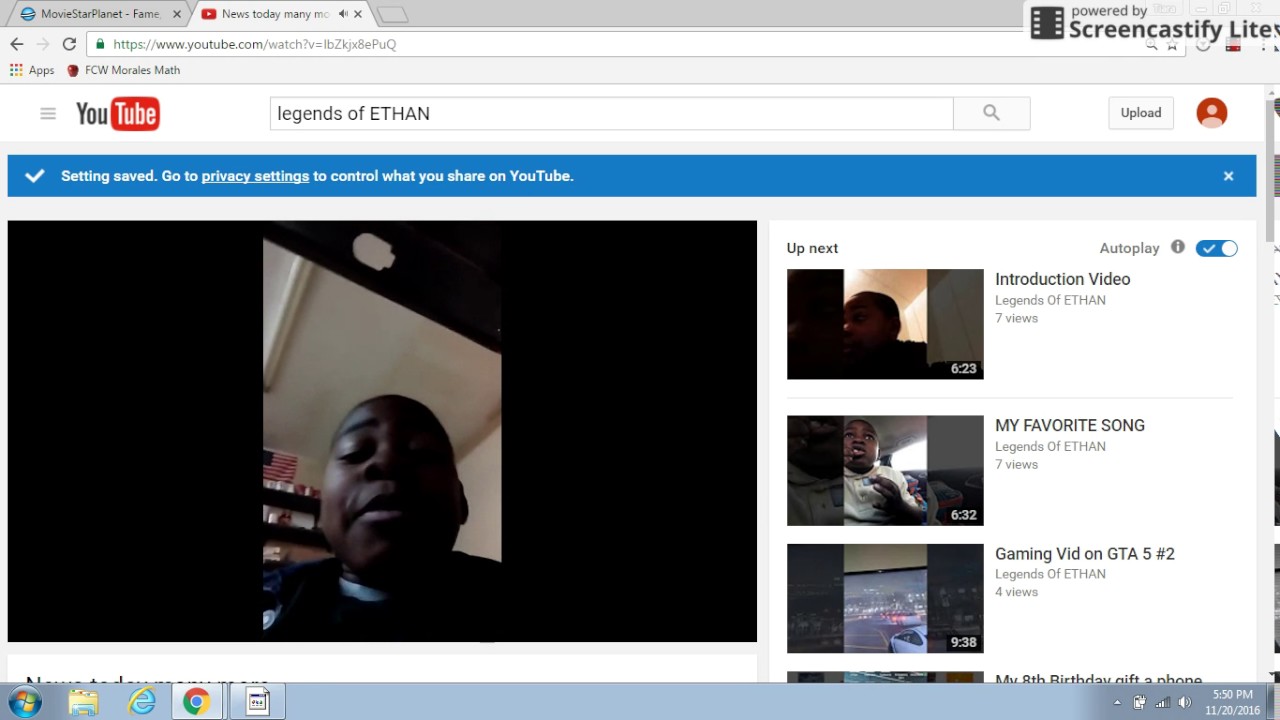The image depicts a YouTube browser page. In the upper left-hand corner, the first tab appears to be labeled "Movie Star Panel," although part of the text is cut off. To the right, there's another tab partially labeled "News Today Mini M," with the rest of the word obscured. Below these tabs, there is a search bar displaying the YouTube URL. 

To the left of the search bar, there are two navigation arrows; a light gray arrow pointing right and one pointing left. Below the search bar, "YouTube" is prominently displayed, adjacent to a hamburger menu icon on the far left, and a search icon labeled "Legends of Ethan" in the middle. On the right side of the search bar are icons for search, upload, and a sparse-looking profile icon.

Spanning across the middle of the image, a blue banner displays a message with a checkmark, reading, "Setting Saved. Go to Privacy Settings to control what you share on YouTube." The phrase "Privacy Settings" is underscored, indicating it is a clickable link.

In the center of the image, there's a picture of a young Black male, showing his face and shoulders. The rest of the image around him is dark and cut off. On the right-hand side of the image, three videos are queued up next for autoplay. At the bottom left corner, five icons are displayed, though their specific functions are not detailed in the description.